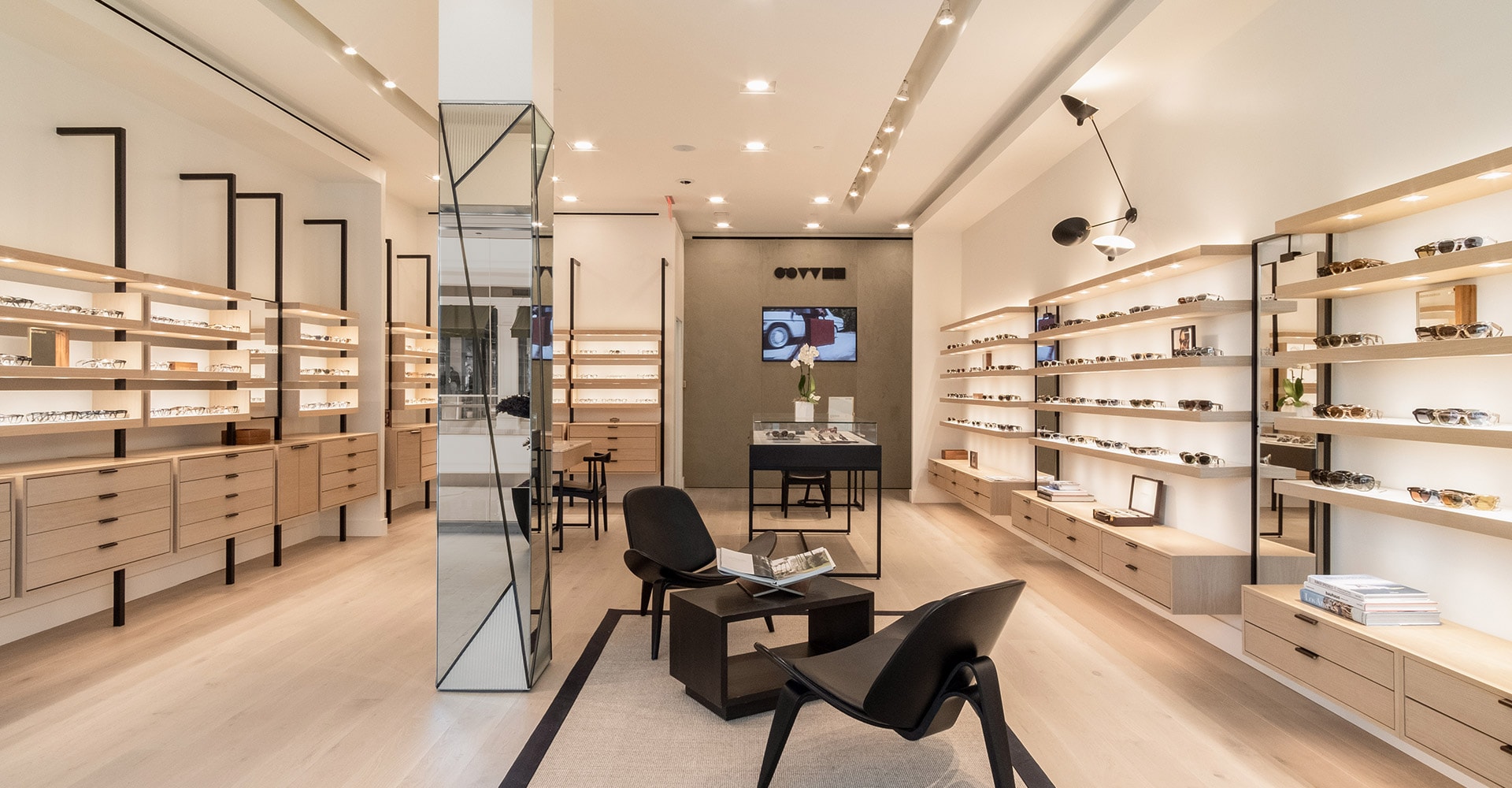The image depicts a brightly lit eyeglass or sunglass store with a light beige interior. On either side of the store, there are several well-lit display shelves filled with various glasses, each shelving unit featuring four to five shelves with drawers or cabinets underneath. These shelves line both the left and right walls, with four rows on each side. Toward the back of the store, a TV screen is mounted on the wall, in front of which sits a display desk showcasing more glasses. A vase of flowers and some objects like a suitcase and book stacks are placed on some of the cabinets. In the foreground, there are two black chairs and a matching black table, which holds an open book on a stand. Additionally, there is a pillar with a mirror wrapped around it, adding to the store's elegant and organized appearance.